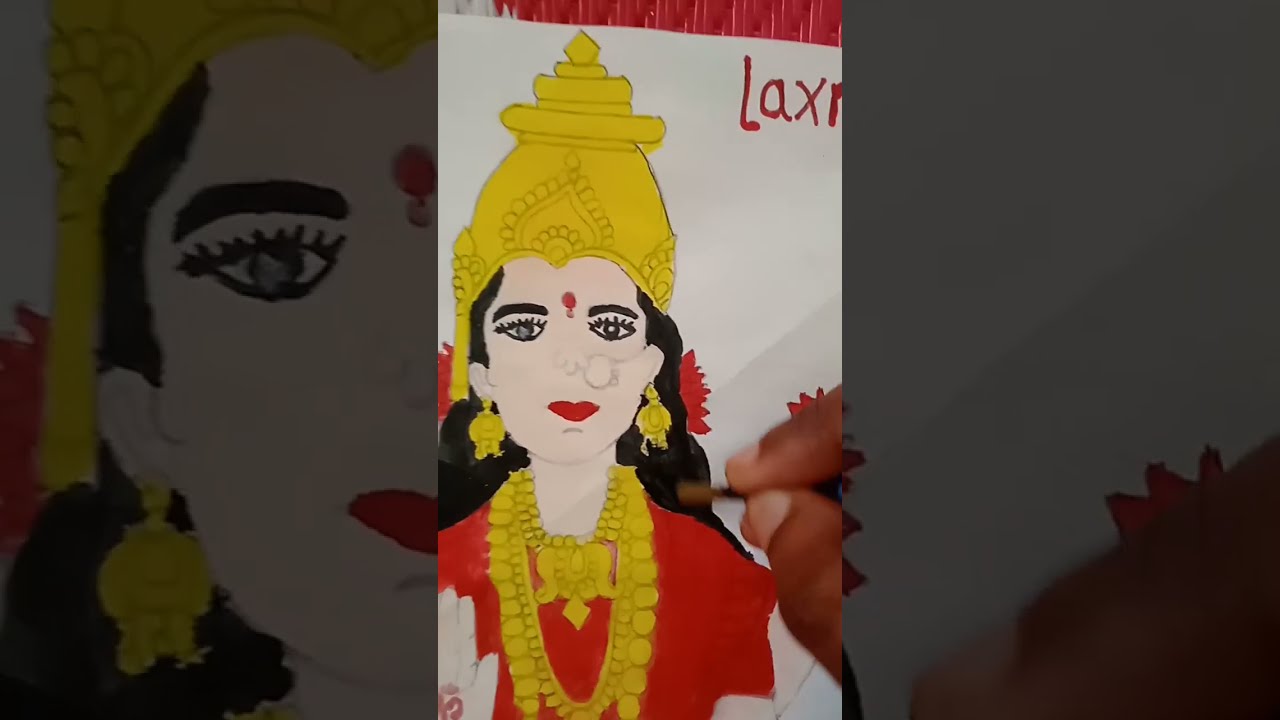The image depicts a detailed sketch of a goddess on white paper. The goddess is adorned with elaborate gold jewelry, including a golden crown with three tiers, gold earrings, and multiple gold necklaces. She is dressed in red garments and has a prominent red dot on her forehead. Her long black hair is being meticulously painted by a pair of dark-skinned fingers holding a paintbrush, emphasizing the ongoing artistic process. The background of the paper remains white, with the partial word "LAX" visible in the top right corner. Surrounding the central image, the left and right vertical sections feature close-up, darkened enlargements of the same sketch, creating a layered, portrait-style presentation.